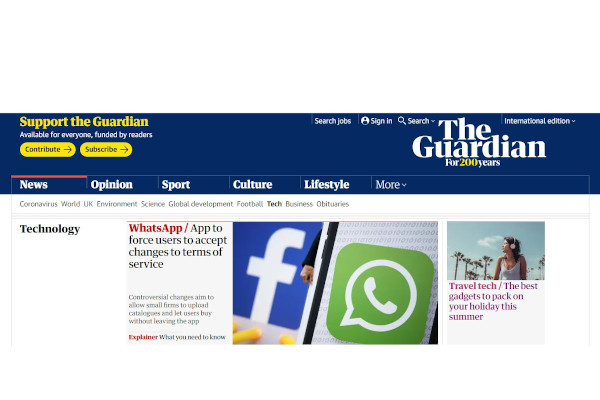Screenshot of The Guardian's website. At the top of the page, the header prominently features the phrase "The Guardian for 200 years" on the right-hand side. On the left, a call to action reads, "Support The Guardian, available for everyone, funded by readers." Below this message, there are two yellow buttons: one labeled "Contribute" and the other "Subscribe." The menu bar beneath the header displays various categories: News, Opinion, Sport, Culture, Lifestyle, and a "More" option. The main headline of the webpage is about technology and states, "WhatsApp app to force users to accept changes," referring to updates in the app's terms of service.